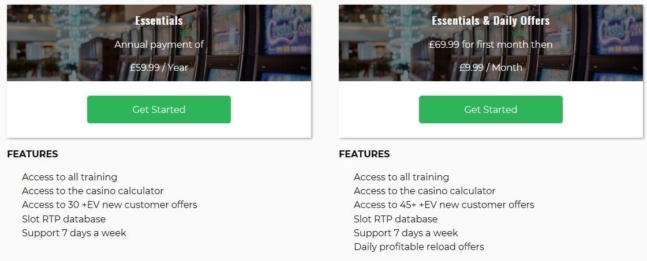On the left side of the image, there's a detailed advertisement for a subscription service. The background features an image of slot machines and a chandelier, adding a touch of opulence and excitement. The text overlay highlights an "Essential Annual" payment plan available for £59.99 per year. Below this information, in a white area, there's a prominent green rectangular button labeled "Get Started." 

Underneath the button, you'll find a list of features included with the subscription:
- Access to all training
- Access to the casino calculator
- Access to over 30 EV new customer offers
- Slot RTP database
- Support available 7 days a week

On the right side of the image, the visual theme with the slot machines is repeated, emphasizing consistency across subscription plans. This section advertises the "Essential and Daily Offer" plan which is priced at £69.99 for the first month and then £9.99 per month thereafter. Again, a white area below the text contains a green rectangular “Get Started” button.

The list of features for this plan includes:
- Access to all training
- Access to the casino calculator
- Access to over 45 EV new customer offers
- Slot RTP database 
- Support available 7 days a week